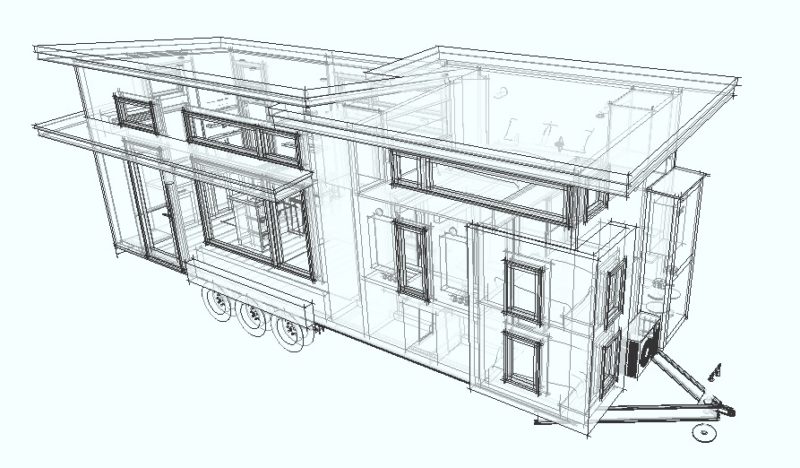This image depicts an architecture-style sketch, potentially AI-generated, of a modern mobile home or trailer. The monochrome illustration, with its transparent, pixelated lines, allows a view of the interior layout. The structure, viewed diagonally, features multiple rectangular windows and is set on three wheels. A triangular hitch at the front indicates the home is designed for mobility. The roof is notably distinctive, with two diagonally aligned panels to facilitate rain runoff. The minimalistic style, characterized by its rectangular form and lack of texture, contributes to its modern aesthetic, suggesting it might be a prefabricated home or building on wheels.